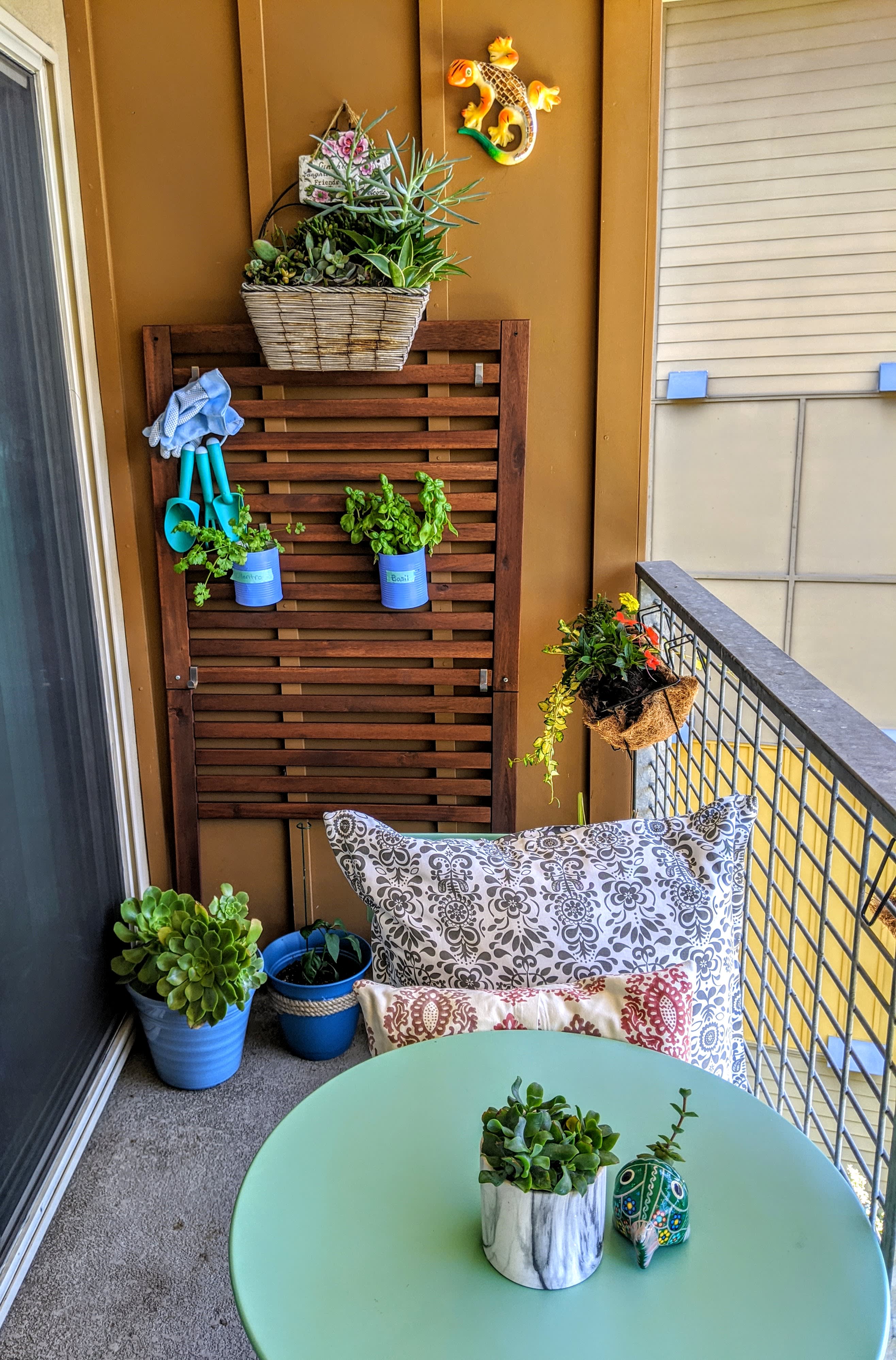This photograph captures a small, vibrant balcony space with a cozy and eclectic mix of decor and gardening elements. Dominating the left side of the image is a sliding glass door equipped with a mesh screen to keep insects out. The backdrop features a mustard-yellow wall adorned with a wooden lattice structure, hosting a variety of plants, light blue gloves, and turquoise gardening tools, including a shovel and rake. On the right, a gray metal fence provides a barrier.

In the middle ground of the image, a mint green circular table is prominently featured. Atop the table rests a white pot with dark blue marbling containing a thriving green succulent. Next to it sits an artistic, green fish-shaped pot with a green plant sprouting from its mouth. A green chair is partially visible, tucked into the table, covered by two elaborate patterned pillows—one primarily gray and the other red.

Adding to the charm, the lattice structure on the back wall supports two purple painted pails labeled with herbs, one visibly marked "basil." Above this, a large brown wicker basket overflows with plants, situated near a decorative sign adorned with pink flowers. An eye-catching yellow gecko adorns the wall, adding a whimsical touch. Finally, the concrete floor supports two more blue pots brimming with plants at the bottom corner near the screen door, while a small artistic snail sculpture on the table holds another succulent in its granite container, completing the verdant, serene setting.